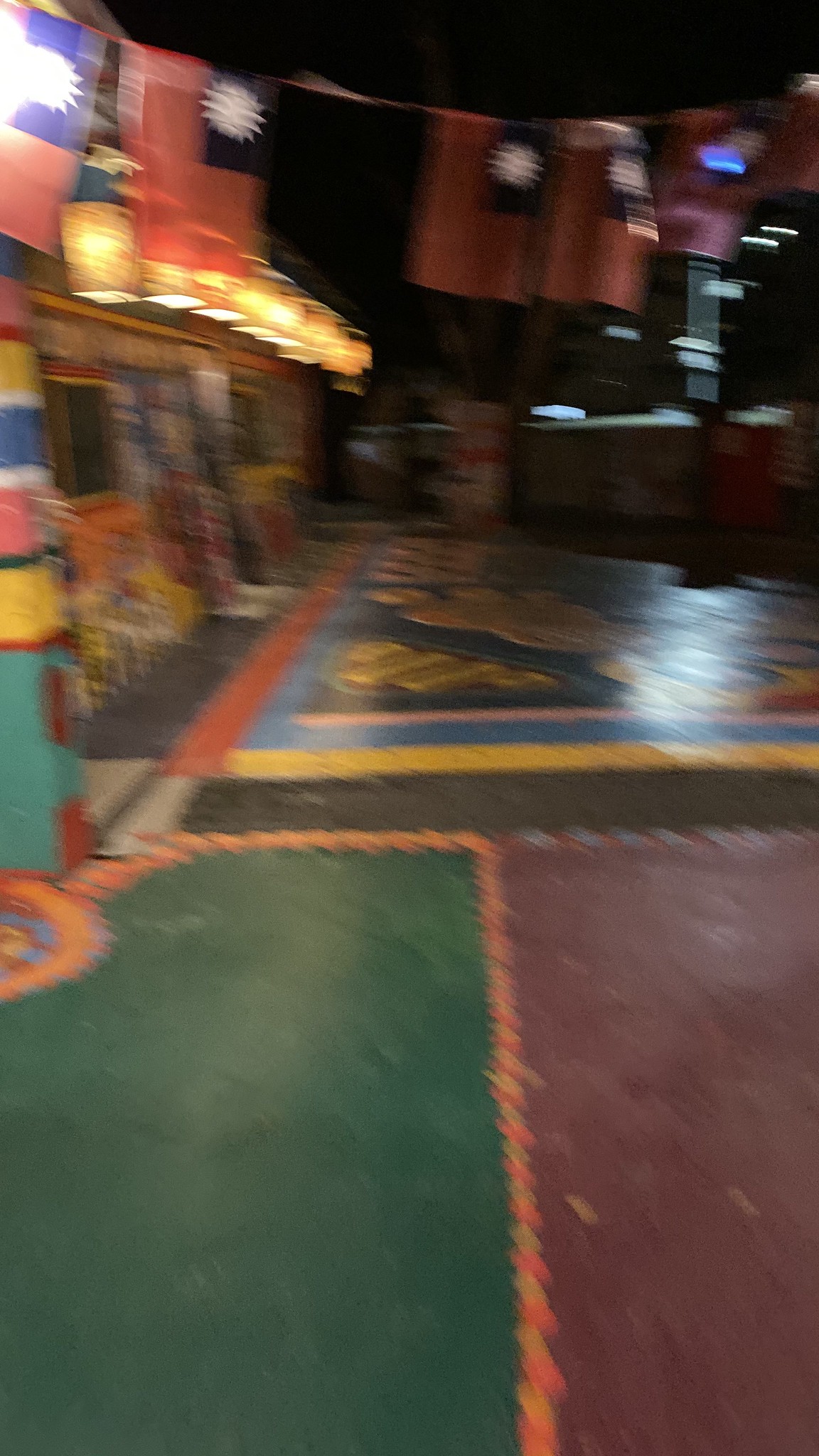The image appears to be taken inside an energetic and vibrant space, possibly a children's playroom, a kid's museum, a party venue, an arcade, or even a bowling alley. The foreground of the picture is dominated by a colorful floor that includes distinct segments with a green and red side, each adorned with orange dots. Adjacent to this, extending across the floor, are additional sections featuring colors like yellow, blue, and orange, intricately decorated with various patterns that might resemble plugs or footprints.

On the right side of the image, a series of lights adds to the vibrant ambiance. These lights stretch from the top right corner downwards towards the center; they could potentially be lanterns or light fixtures with unique tops. Below these lights, near the bottom edge of the image, there appear to be packages or gifts along the wall, contributing to the festive atmosphere. 

The ceiling is also decorated, sporting orange flags and blue flags, each with white starburst patterns. Additional light sources can be spotted towards the background, though the exact details remain indistinct due to the blurriness of the image. Overall, the scene conveys a lively and celebratory environment, ideal for children or family activities.